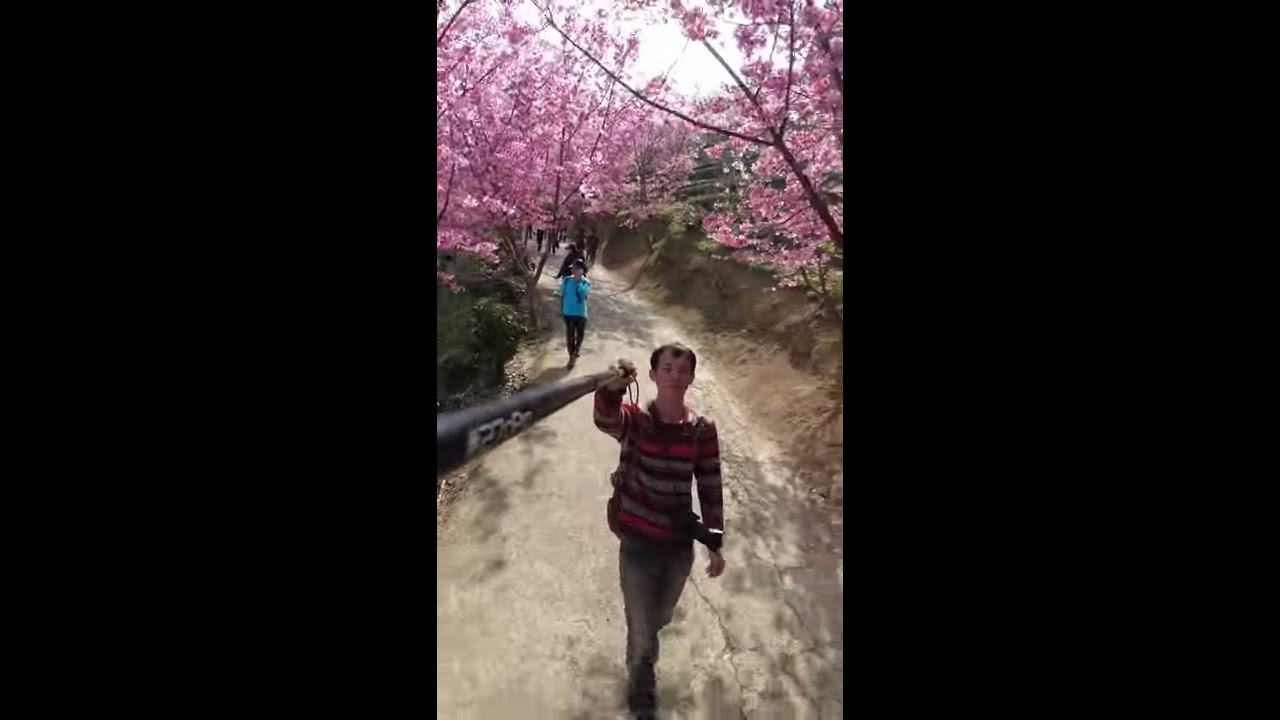The wide rectangular image centers on a tall, rectangular photograph capturing a young person hiking down a light gray, paved trail, taking a selfie. The background to the left and right of the photograph is entirely black. The trail originates from the bottom right and narrows as it heads towards the top left corner. 

The focal point of the image is the young hiker, who is wearing a black, gray, and red striped sweatshirt with gray jeans. He is holding a selfie stick in his left hand, which extends towards the left side of the image. Additionally, he carries a large photography camera on a strap over his shoulder, resting at his waist. 

On the right side of the trail is a wall of brown dirt seamlessly transitioning into a grassy area. A large cherry blossom tree, adorned with vivid pink blooms, grows from this wall. The left side of the trail is flanked by lush greenery and dark green bushes interspersed with more cherry blossom trees. 

In the background, several people can be seen walking along the pathway, including a woman in a bright blue top and a group of individuals dressed in black, all seemingly enjoying the scenic hike amidst the blooming cherry blossoms.